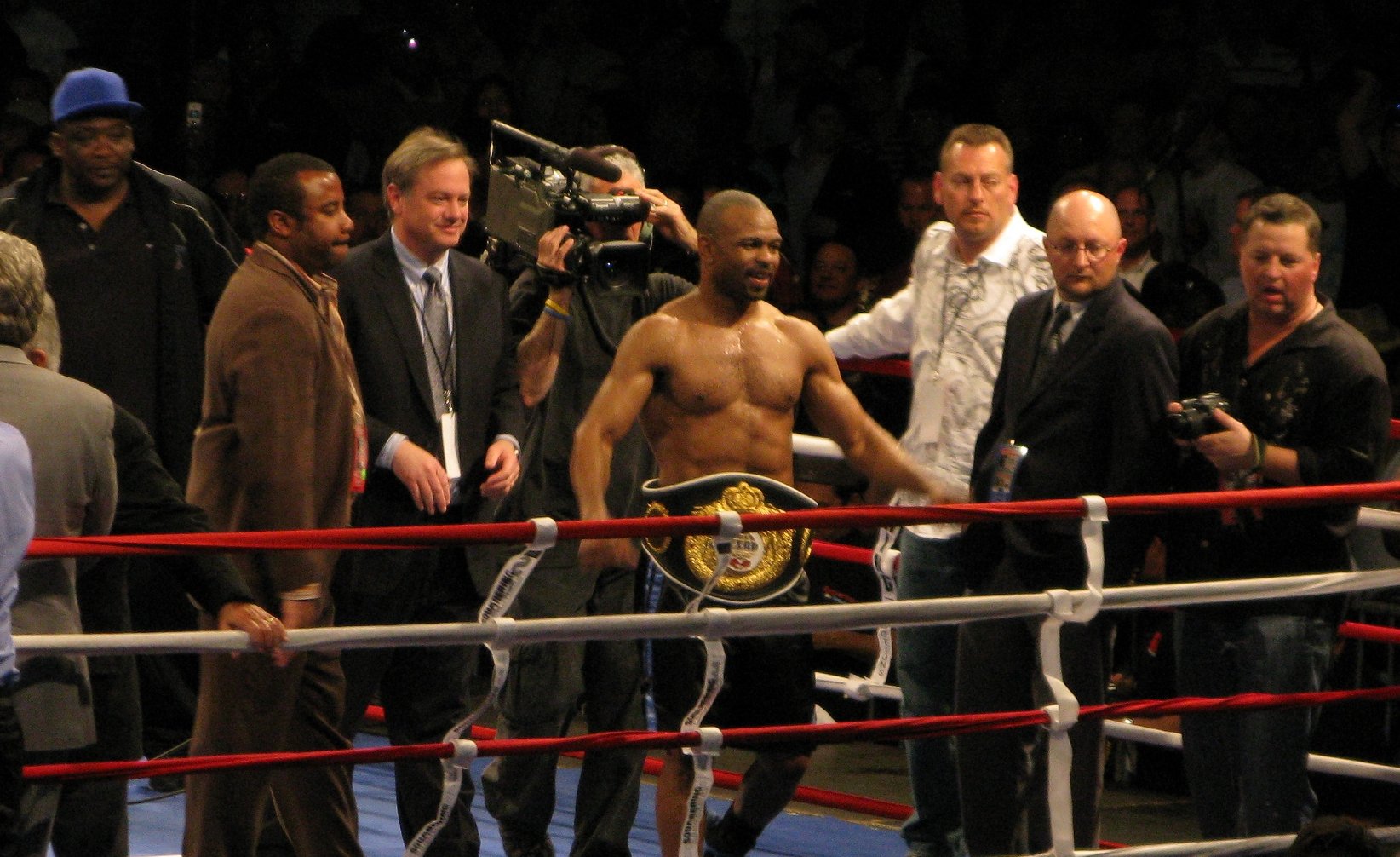The image captures the triumphant moment at the end of a boxing match. In the center of the ring stands a victorious boxer, wearing dark trunks with blue stripes on the sides, appearing sweaty and exhilarated. He proudly dons a large, ornate championship belt adorned with a golden seal featuring text, a testament to his hard-earned victory. His arms are outstretched on the ropes, and he appears to be smiling, though the distance from the camera makes it difficult to discern his exact expression.

Surrounding him, the atmosphere is bustling with activity. Directly behind the boxer, a cameraman holds a large camera, partially obscuring his face. He is dressed in jeans and a dark shirt, contributing to the documentation of the moment. To the left of the boxer, three men stand: one in a white shirt, another in a black suit, and the third in a dark button-up shirt, gazing into the distance. On the right side, three more men are present: one in a dark suit with a bluish undershirt, another in a brown suit, and a man wearing a hat and dark polo shirt, all seemingly focused on a common point of interest.

Adding to the vibrant scene, the edges of the ring are outlined with blue and white ropes, and the background is filled with the excited buzz of a crowd witnessing the aftermath of the match. The boxer encapsulates the moment of glory, surrounded by people who share in his triumphant energy.